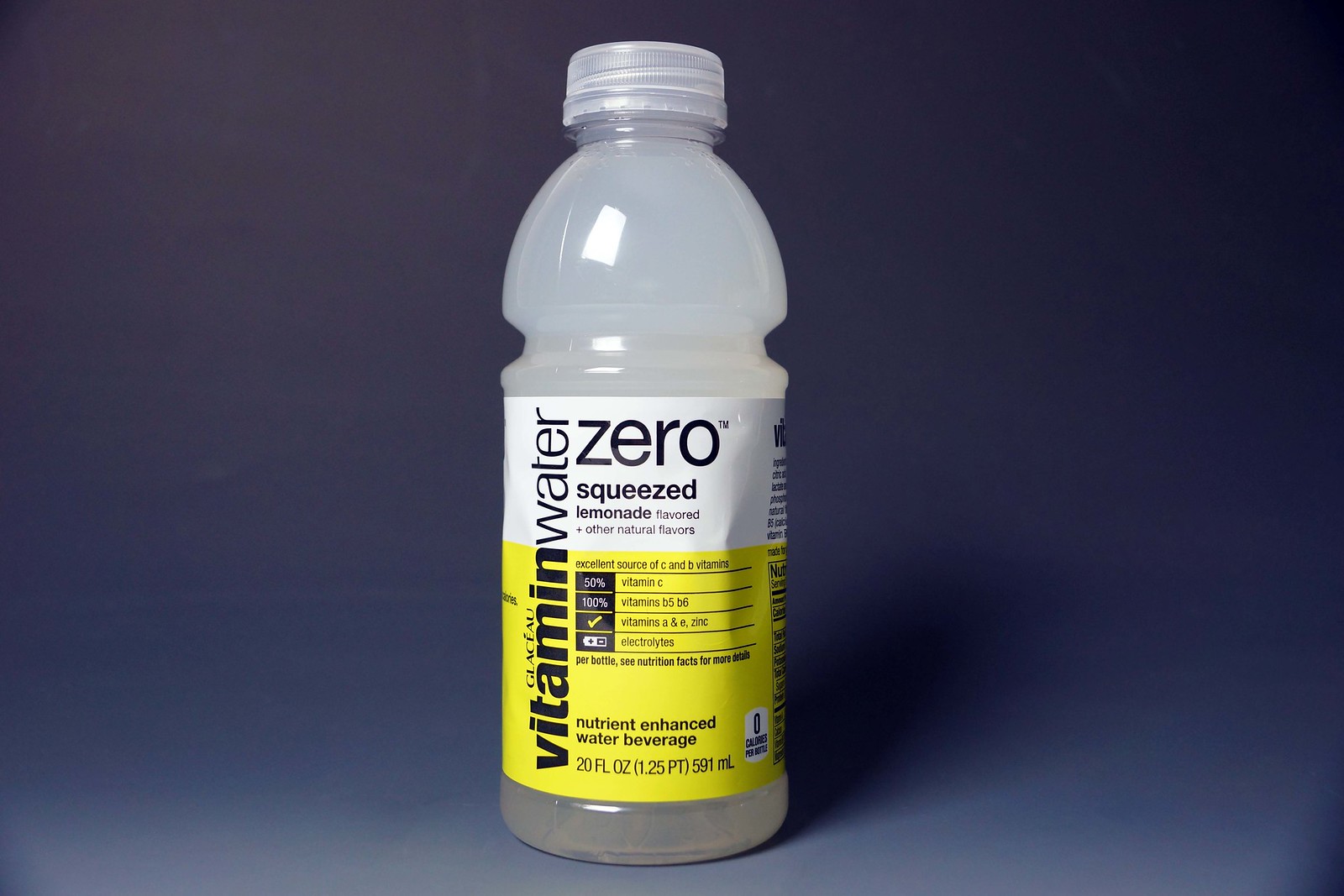The image features a bottle of Vitamin Water positioned against a bluish background and resting on a flat surface. Light illuminates the front of the bottle, casting a distinct shadow behind it. The bottle's label is predominantly white at the top and yellow at the bottom, with the words "Vitamin Water" printed in a vertical orientation. The upper white section of the label details the flavor as "Zero Squeeze Lemonade" followed by the phrase "plus other natural flavors" and additional smaller text. The liquid inside the bottle is opaque and white, rendering it non-translucent. There is a noticeable white area on the surface near the bottom of the image, slightly away from the bottle.